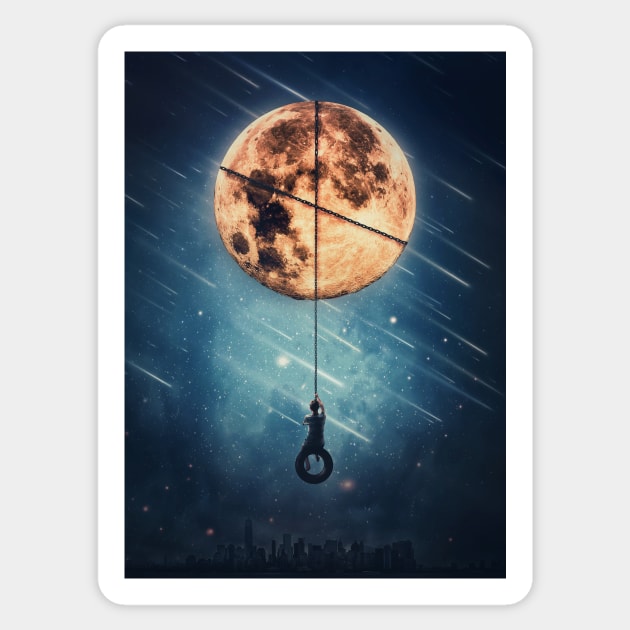In this fantastical artwork, a large, bright orange-and-black moon dominates the scene, radiating a soft glow against a dark blue night sky. Enshrouded by a black chain, the moon has one chain wrapping around it horizontally and another extending vertically down the center. Hanging from this vertical chain, a boy sits atop a rubber tire swing, his back facing the viewer. The sky is adorned with shooting stars and streaks of light that travel diagonally across the image, lending a sense of motion. Below, a dimly lit cityscape silhouette, possibly resembling New York, stretches across the lower part of the image. The skyline features prominent skyscrapers centrally and smaller buildings towards the edges, blending into flatter land. The scene evokes a dreamlike blend of whimsy and serenity.